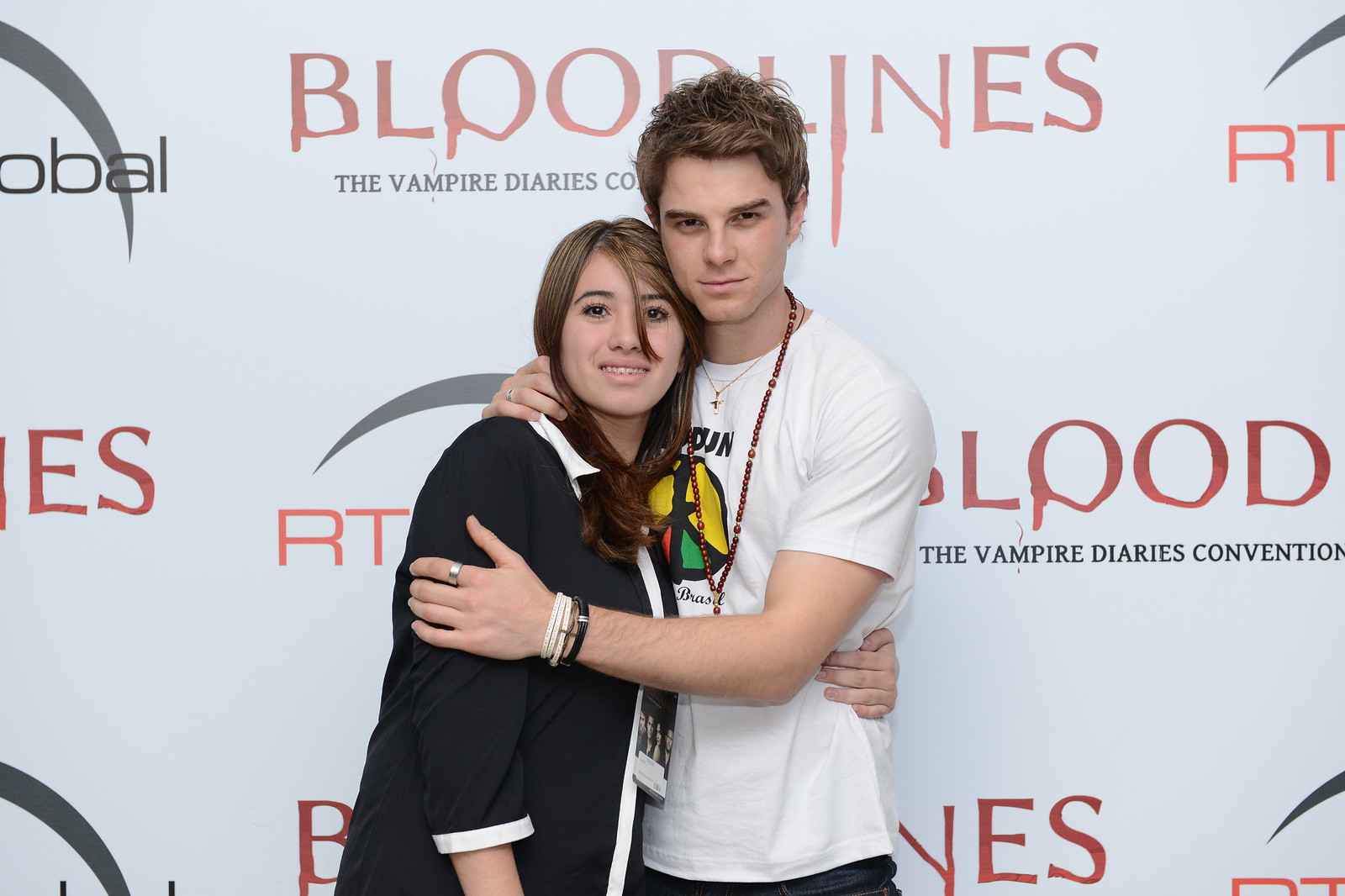In this detailed photograph, set against a backdrop emblazoned with the word "BLOODLINES" in red and "The Vampire Diaries Convention" in grey, two young adults are captured in a warm embrace. The backdrop, designed specifically for the convention, repeats the words prominently, creating an unmistakable theme. 

The image centers on a young man and woman, both in their 20s, standing closely together. The man, positioned on the right, is notably taller with short spiky brown hair. He dons a white t-shirt adorned with a red, yellow, and green graphic logo. His accessories include multiple bracelets, a ring on his index finger, a necklace, and a lanyard, adding to his casual convention look. His facial expression is serious, contrasting with his companion's cheerful demeanor.

The young woman, standing to his left, smiles brightly, showcasing her braces. Her long brown hair cascades around her face, and she leans into the man, her arm wrapped securely around his waist while the other arm hangs by her side. She is dressed in a black jacket over a white shirt, which gives her outfit a layered appearance.

Together, they face the camera, creating a candid and affectionate moment against the vibrant, thematic backdrop of the Vampire Diaries Convention.